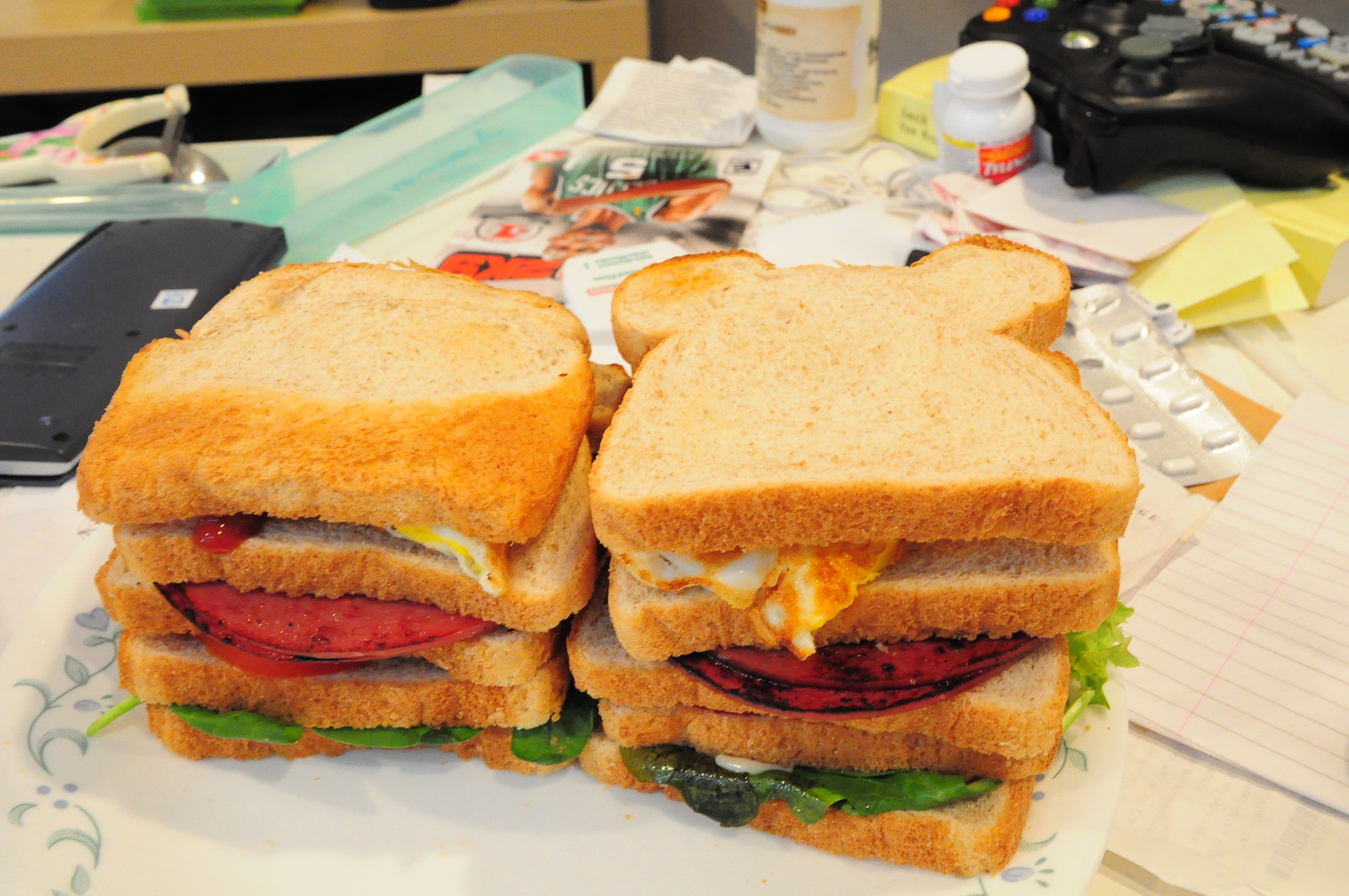A well-lit indoor photograph captures a cluttered desk or table, topped with a white tablecloth featuring subtle floral patterns. The central focus is on two towering sandwiches composed of neatly stacked layers of ingredients on lightly toasted white bread with golden crusts. Each sandwich features approximately eight slices of bread, each holding different layers like fried bologna, eggs, lettuce, tomato, and a hint of mayonnaise. Surrounding this gastronomic spectacle, the tabletop is scattered with a variety of items: to the top right, a black video game controller and a matching TV remote sit adjacent; nearby is a white bottle with an orange Tylenol label. Among the clutter are loose pills, an upside-down black calculator, a long blue plastic tube, and scattered papers, including yellow and white sheets. The general chaos of the desk contrasts the orderly arrangement of the sandwich layers, making for a visually compelling scene.